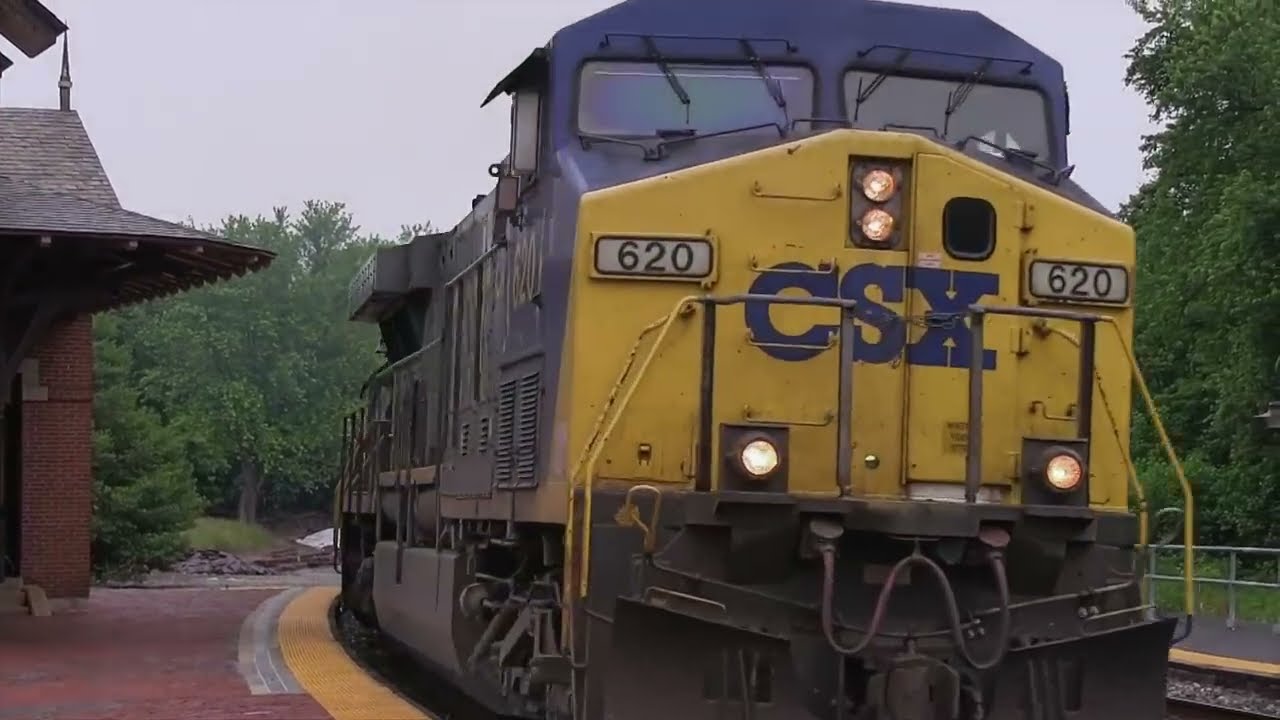The image captures a bustling train station on a cloudy, possibly late afternoon. Dominating the scene are multiple train tracks: one curves left towards the background, another parallel track follows a similar path, and a third rail line veers off to the right. Nestled among these tracks is a cargo boxcar, likely the caboose, identifiable by its square shape and the absence of a visible locomotive or driver. Notably, a stick with a red cloth is fixed to the back of the train. In the gap between the center and right tracks, a collection of black rails or guards lies scattered on the gravel. 

Near the foreground, a ladder leaning against steel beams hints at a maintenance area. On the left side, there's a train platform equipped with stoplights and a digital sign, though the exact text is unreadable from this distance. Both sides of the scene are bordered by lush, green tree lines, suggesting it's summer. The right side appears to rise into a hill. This intricate interplay of man-made and natural elements, set against a hazy, potentially sunset sky, creates a vivid snapshot of a train station in operation.